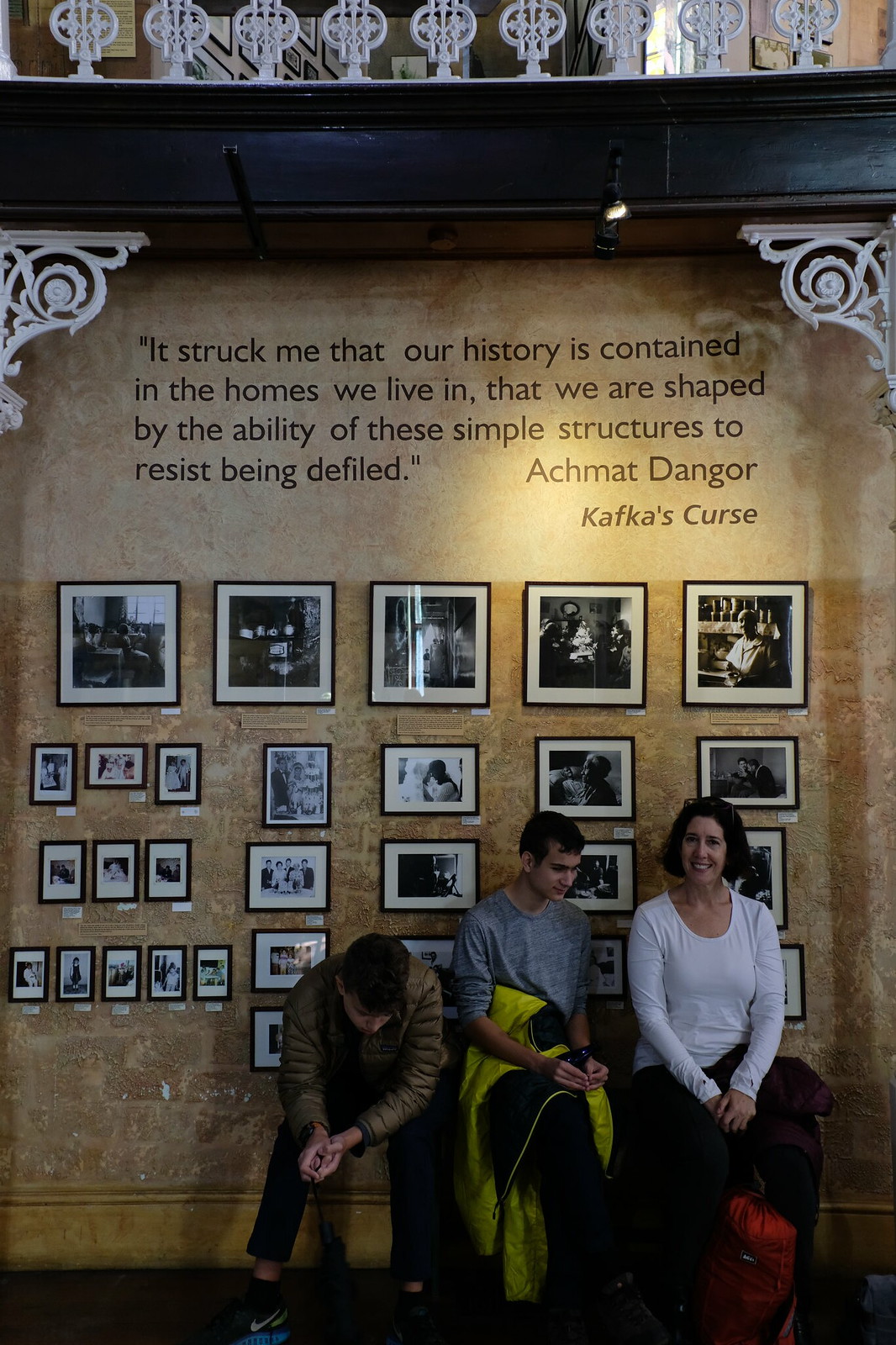In the foreground of this portrait-oriented image, seated towards the lower right, are three individuals that appear to be a mother and her two sons. The woman on the far right is the only one looking at the camera. She is seated, wearing a white top paired with black pants, exuding a motherly appearance. She has a red duffel bag at her feet, suggesting they might be traveling. To her left is a young boy, possibly in his late teens, wearing a gray t-shirt and holding a yellow and black jacket in his lap. He is comfortably facing the mother. Further to the left is another boy, who seems bored and is looking down at the ground. He is dressed in a brown jacket, black pants, and Nike shoes.

They are seated in front of a cream-colored wall adorned with rows and columns of framed black and white photographs. At the top of the wall is a quote attributed to Akhmat Dangor, specifically from "Kafka’s Curse." The wall has white border details and architectural elements at the top, adding a classical touch to the setting. The overall composition of the image captures these three individuals posed against this intricately decorated backdrop, blending a sense of personal and historical narrative.